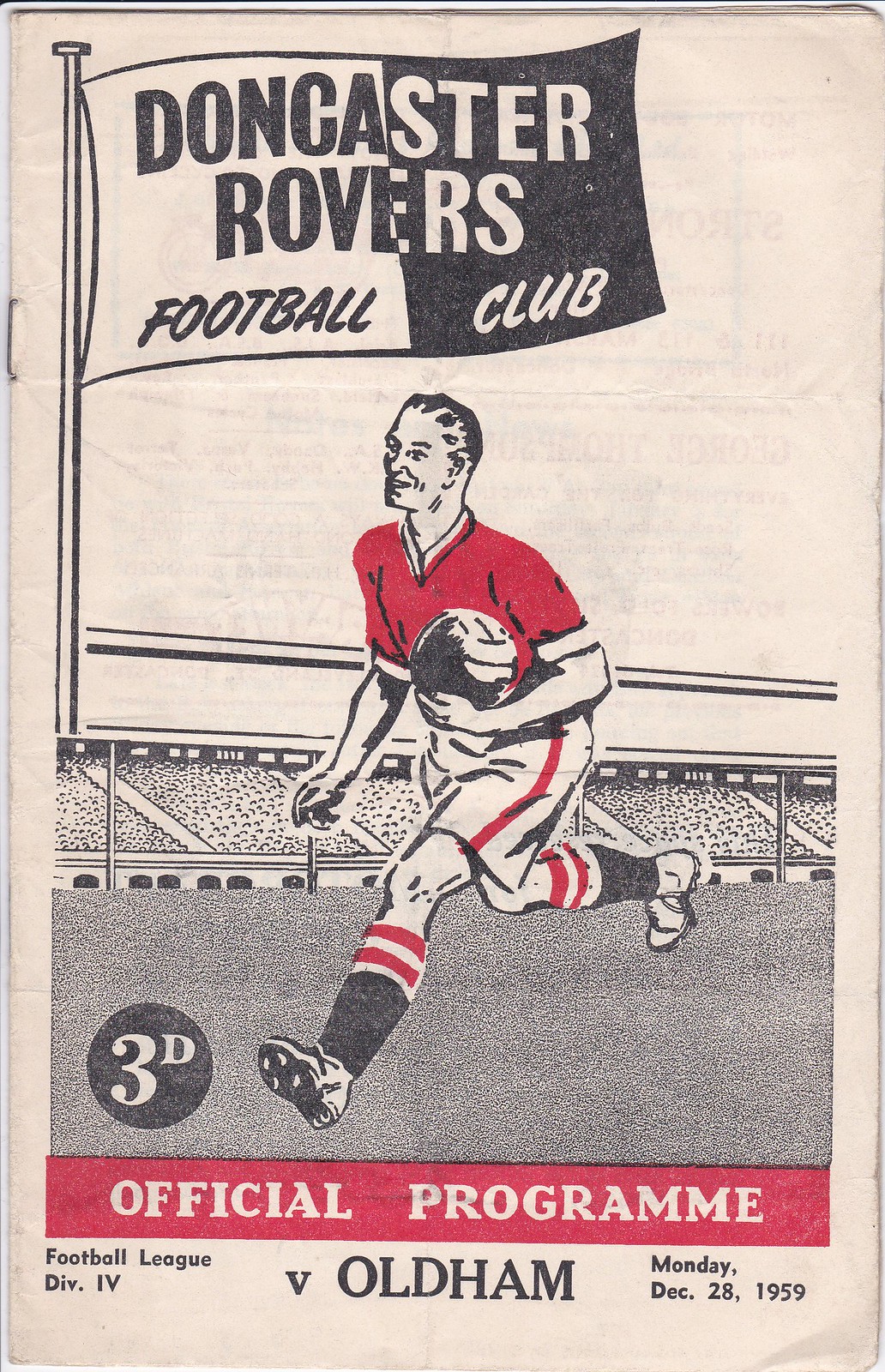This portrait-format illustration appears to be an old, aged magazine cover or a piece of marketing material for a football program. The background is a pinkish cream color. In the upper left-hand corner, a flag waves with the text "Doncaster Rovers Football Club," presented in a black and white split, reversed on either side. 

Central to the image is a detailed drawing of a man seen from a side angle, possibly running. He has a red short-sleeve v-neck shirt, and holds a soccer ball in his left hand close to his chest. He wears white shorts with a red stripe down the side and knee-high socks featuring alternating red and white stripes at the top. His black socks extend from his calf down to his ankles where he wears white cleats.

In the backdrop, a stadium with closely packed crowds is depicted with black dots representing the audience and the grass. Across the bottom is a red banner with white text reading "Official Program". Below that, in black text, it says "Football League Division 4 V Oldham, Monday, December 28th, 1959."